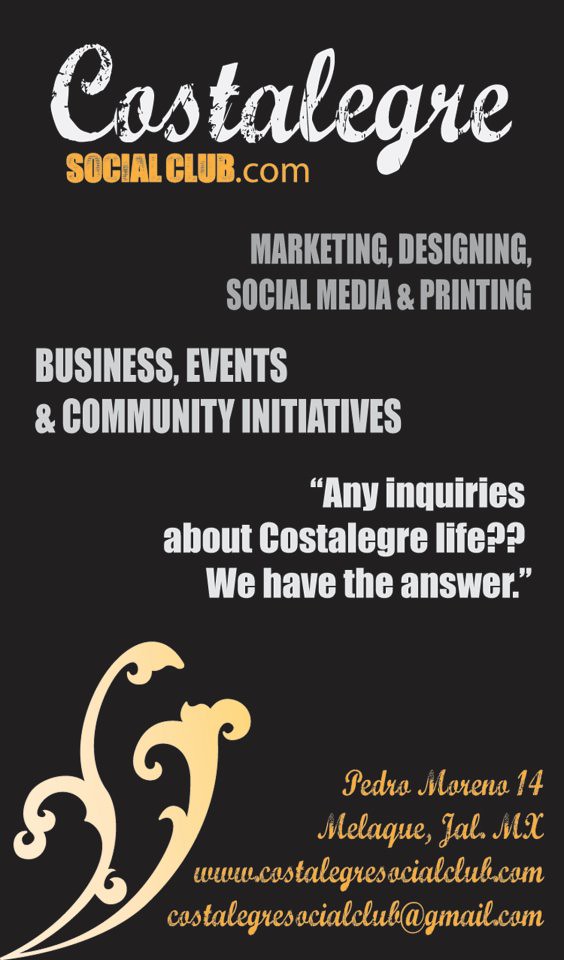The image is a poster or advertisement that promotes the "Costa Ligre Social Club." The main title, "Costa Ligre," is displayed in gold script-like text with "Social Club" written beneath it in white. The poster details the club's services, including Marketing, Designing, Social Media, and Printing, as well as Business Events and Community Initiatives, all written in gray. It also emphasizes their motto in white: "Any inquiries about Costa Ligre life? We have the answer." Additionally, the bottom corner features a decorative white and gold leaf or floral design and provides the contact information, including a street address, website (www.CostaLigreSocialClub.com), and email address (CostaLigreSocialClub@gmail.com), all in script. The colors featured prominently throughout the poster are black, white, gold, tannish, and gray, with a clear and well-spaced layout that makes the information easy to read. The setting and overall style suggest this is a professional advertisement for a marketing and community-focused organization.